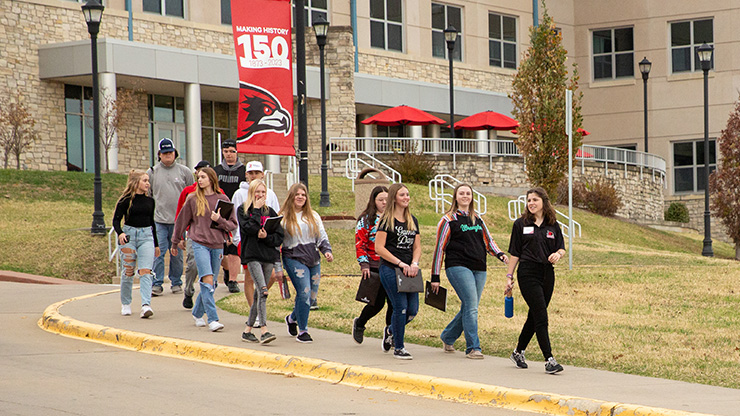The photograph showcases a group of high school students casually exiting a high school building, characterized by its non-uniform beige stone masonry and a canopy over several windows. The scene features students walking down a curved sidewalk that leads from the building, which has a patio area outfitted with tables and red umbrellas. A black lamppost, adorned with a vertical banner proclaiming "Making History 150 Years: 1873 to 2023," is also visible. Among the dozen students, a majority are females, notably four with fashionable, torn-knee jeans. The males in the background, totaling around four, are wearing baseball caps and a mix of casual attire, including sweatshirts and T-shirts. The female at the forefront, possibly a teacher, identifiable by her name tag and attire of black shirt and pants, wields a water bottle. The students appear cheerful and engaged, conspicuously carrying minimal books or school bags. The backdrop includes a grassy area and several tall black lampposts with traditional lanterns, enhancing the picturesque setting of this high school as students conclude their day.